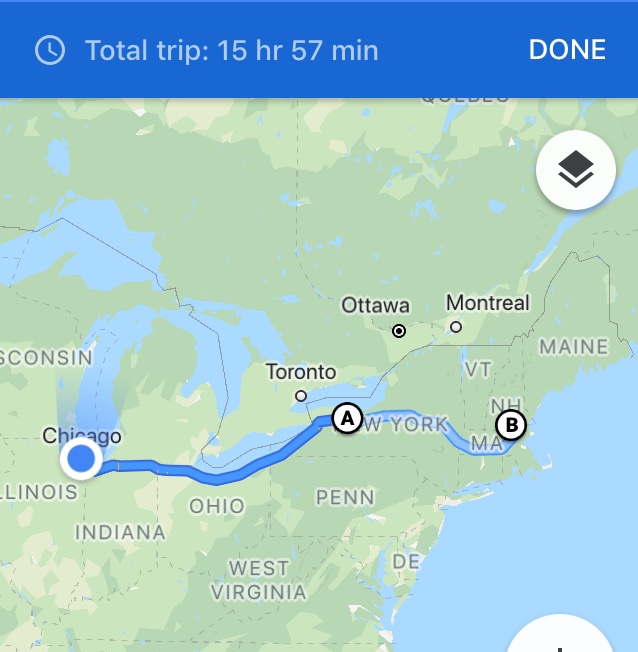This screen capture displays a partial view of the East Coast of the United States on a map. At the top of the image, a blue strip with light blue font reads, "Total trip: 15 hours 57 minutes," alongside a white font label reading, "Done." The map features green-colored cartography, including the states of Maine, Vermont, New Hampshire, Massachusetts, New York, Pennsylvania, Delaware, West Virginia, Ohio, Indiana, Illinois, and Wisconsin. Additionally, it shows parts of Canada, including the cities of Montreal, Ottawa, and Toronto. A segment of the blue ocean is also visible. Each state name appears in dark gray text, while the Canadian cities are labeled in black. Overlaying the map, there is a white circular icon containing a black square in the center, which presumably represents a user interface element.